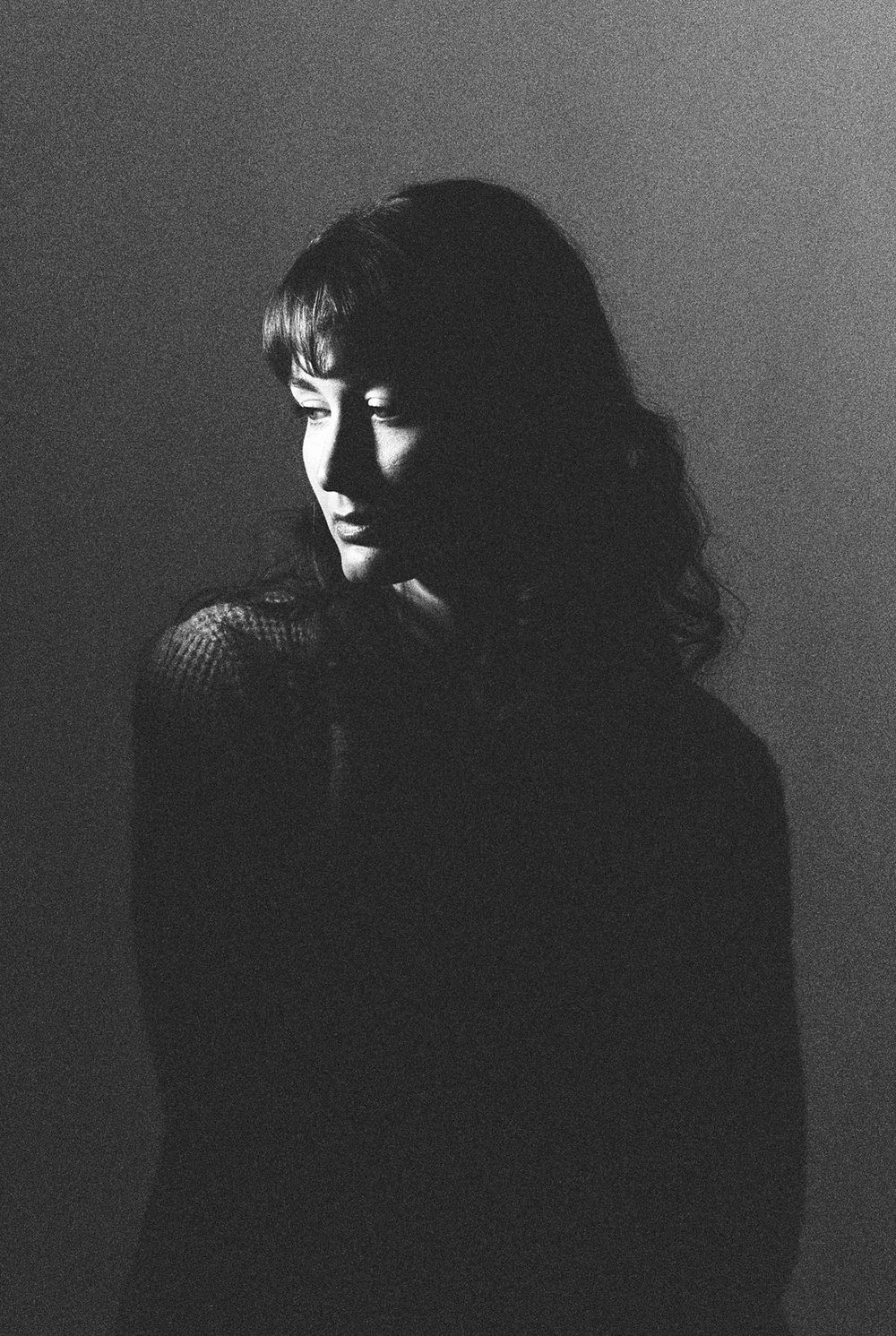This monochromatic photograph captures a dramatic and emotional portrait of a young woman with a forlorn expression. The black-and-white image features strong contrasts and textures, highlighting her dark shoulder-length hair with bangs. The woman is the central focus, with light coming from the left, casting a shadow to the right side of the frame. Her head is tilted slightly to the left, and she appears to be looking down, her expression suggesting sadness or contemplation. Her left shoulder is slightly higher, and she seems to be in a knit material, though specific details of the attire are obscured by the heavy chiaroscuro effect. The light accentuates her face while the rest of her form remains in a shadowy silhouette, set against a slightly lighter but still dark background. The photograph possesses a grainy texture, adding to the overall somber and reflective mood of the composition.